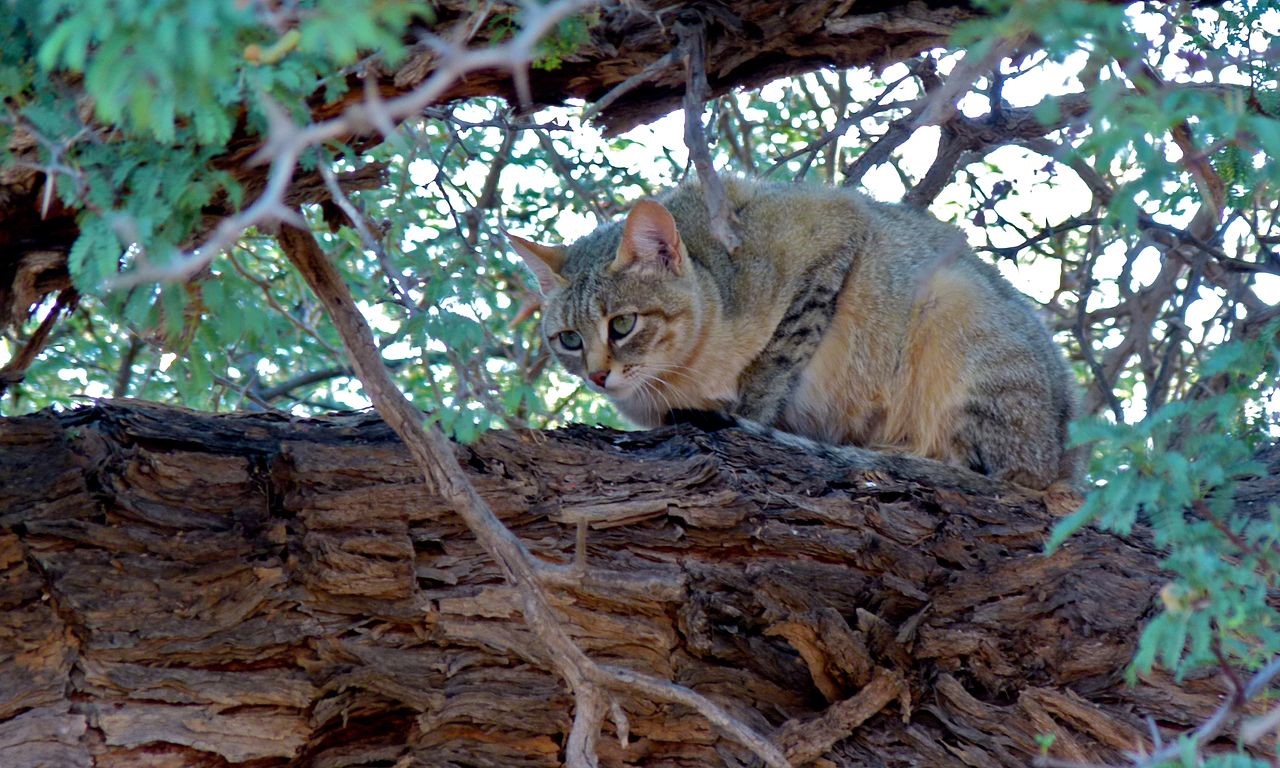In this outdoor photograph, the focal point is a well-fed, exotic-looking cat perched high on a thick, dark brown tree branch that stretches horizontally across the bottom of the image. The cat, centrally positioned but slightly towards the right, is crouched down as if hiding. Its coat features several shades of brown and tan, complemented by darker black and gray tabby stripes, while its stomach is noticeably lighter. The cat’s head is a brownish-gray with darker patches, pink perked ears, light blue to gray-green eyes, and distinct white whiskers. Surrounding the scene are lush green leaves covering numerous tree branches, with glimpses of the sky shining through, contributing to the natural, serene backdrop. The interplay of green leaves and various shades of brown from the tree and cat creates a harmonious color palette, highlighting the serene beauty of the nature scene.